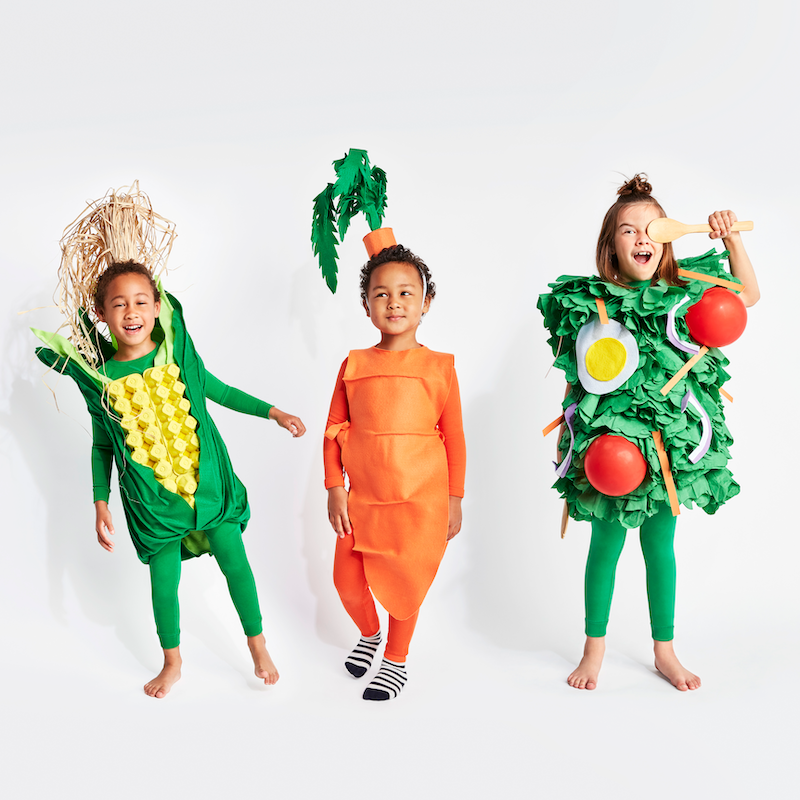In this delightful stock photo, three children are dressed in vibrant Halloween costumes themed after healthy foods, arranged against a plain white background. Starting from the left, a child of color with medium complexion and short, curly hair wears an elaborate corncob costume. This outfit features a 3D green corn husk tunic over green elastic leggings, topped with a brown raffia hat mimicking corn husk tops. The middle child, also a child of color with similar features, suggesting they might be twins, is dressed as a vibrant carrot. This costume comprises an orange tunic that tapers down like a carrot, complemented by a green leafy cap and finished with distinctive black and white striped socks. To the right, a girl with reddish-auburn hair pulled into a small bun is adorably dressed as a whimsical salad. Her costume is adorned with various salad leaves, shreds of carrots, cabbage, and onions, along with 3D egg and tomato decorations. She wears green leggings and is barefoot, smiling while playfully covering one eye with a wooden spoon. All three children, approximately six to eight years old, look charming and cheerful in their imaginative, food-themed Halloween costumes.